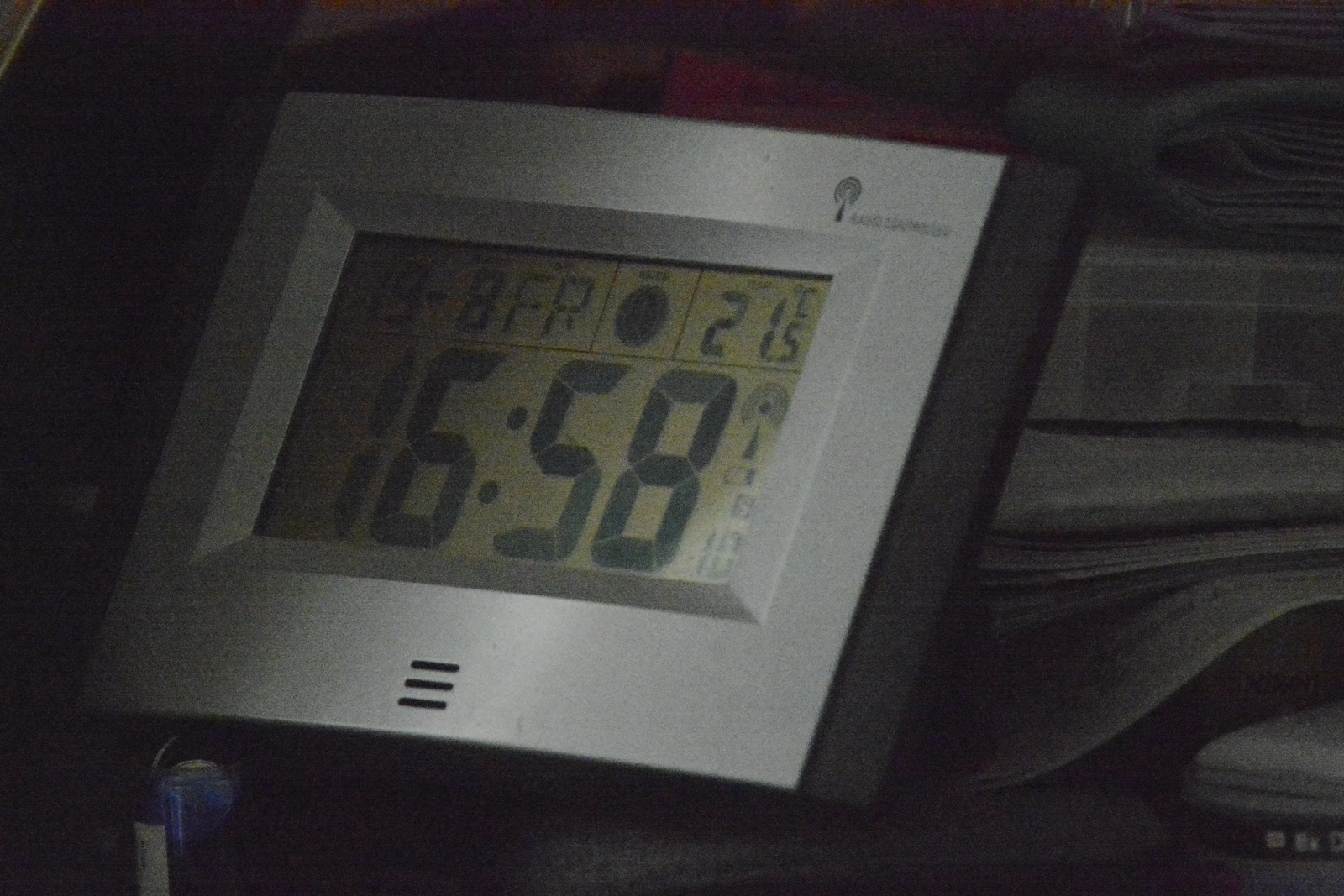The image depicts a digital travel alarm clock leaning against a stack of newspapers in a dimly lit setting, possibly on a cluttered desk. The clock, which has a square design, features a silver metal frame surrounded by a black plastic border. Its display is a pale yellow-green color, showing the time as 16:58 in black numerals. Above the time, the day is indicated as Friday with the date shown as 19-8, likely representing August 19th. The temperature reading is displayed as 21.5 degrees Celsius. The clock's background has three lines of perforations that seem to serve as a speaker. There is also an illegible brand name located in the upper right corner of the display area.